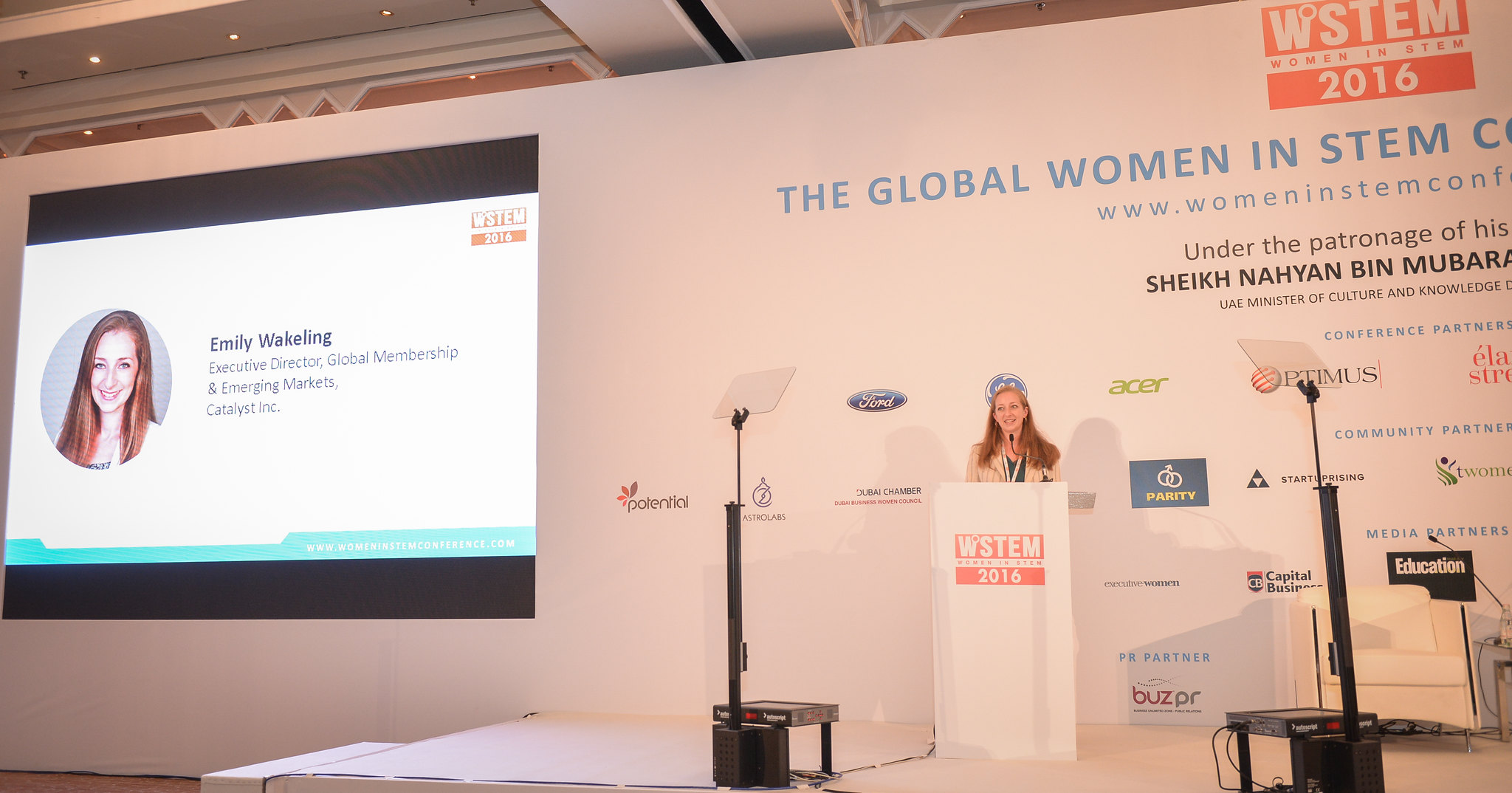The photograph captures a woman standing behind a white podium on a stage, giving a presentation at the "Global Women in STEM 2016" conference, held under the patronage of Sheikh Nayan Bin Mubarak. The stage is illuminated with various lights and equipped with microphones. Behind the speaker, there is a large screen or temporary wall displaying the event's logo and title, "WSTEM: Women in STEM 2016." To the left of the woman, a slide is projected that identifies her as Emily Wakeling, the Executive Director of Global Membership and Emerging Markets for Catalyst Incorporated. Emily is dressed in a black shirt paired with a coat and has long red hair that extends slightly past her shoulders. The projected slide includes a circular picture of her smiling.